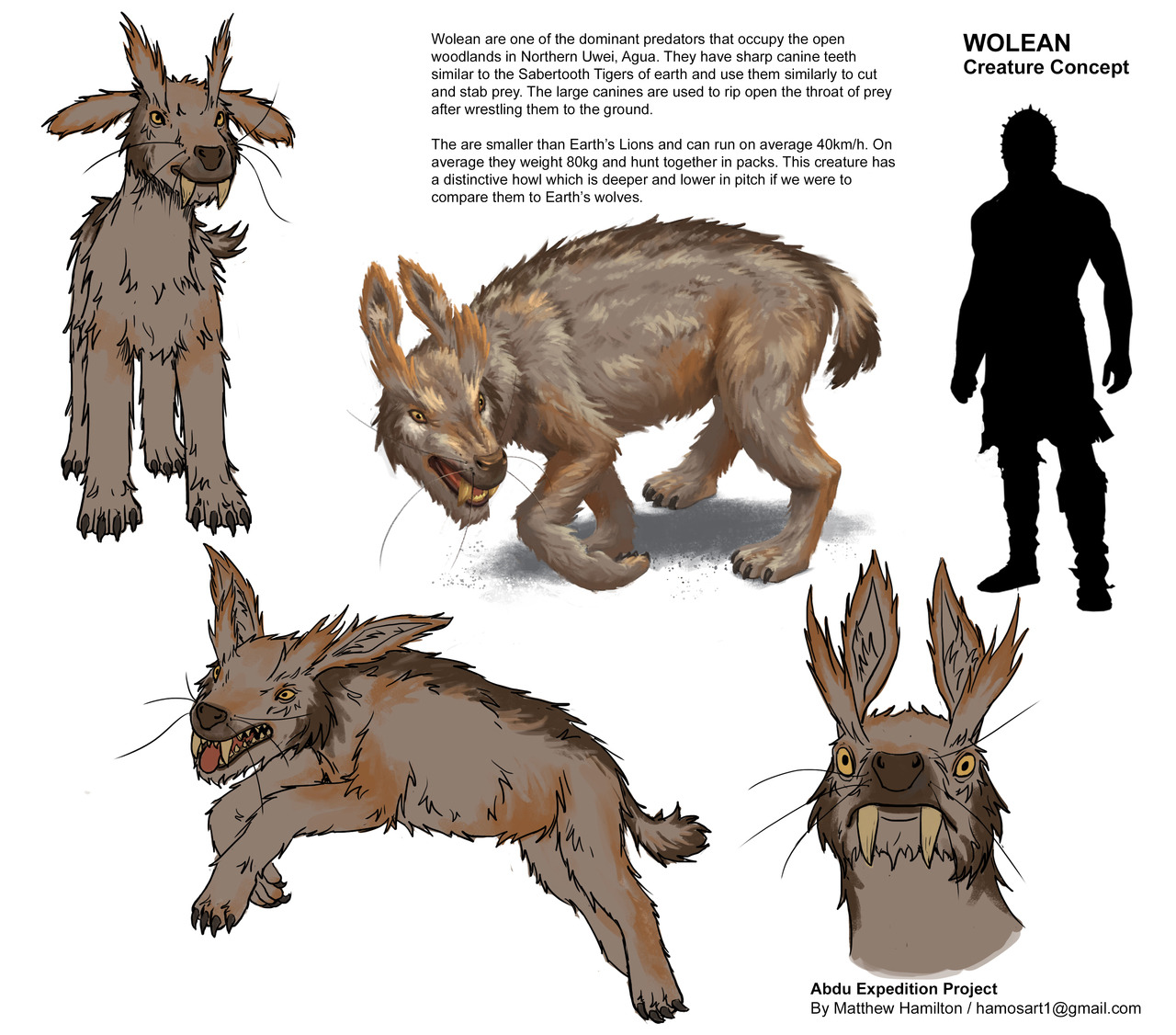The illustration series titled "Wolian Creature Concept," created by Matthew Hamilton and part of the Abdu Expedition Project, depicts a fantastical creature that appears to be a hybrid between a dog, rabbit, wolf, and goat. The Wolian is predominantly brown with a wolf-like snout, two prominent fangs, long ears, and tufts of hair resembling billy goat horns. The images, presented in a color square format, include views of the Wolian in different poses such as running, standing still, and close-ups of its face. A black silhouette of a person is included for scale. Text accompanying the illustrations indicates that Wolians are dominant predators in the open woodlands of northern Uwei, Agua. The concept blends cartoony and 3D elements to vividly bring this imaginative creature to life.